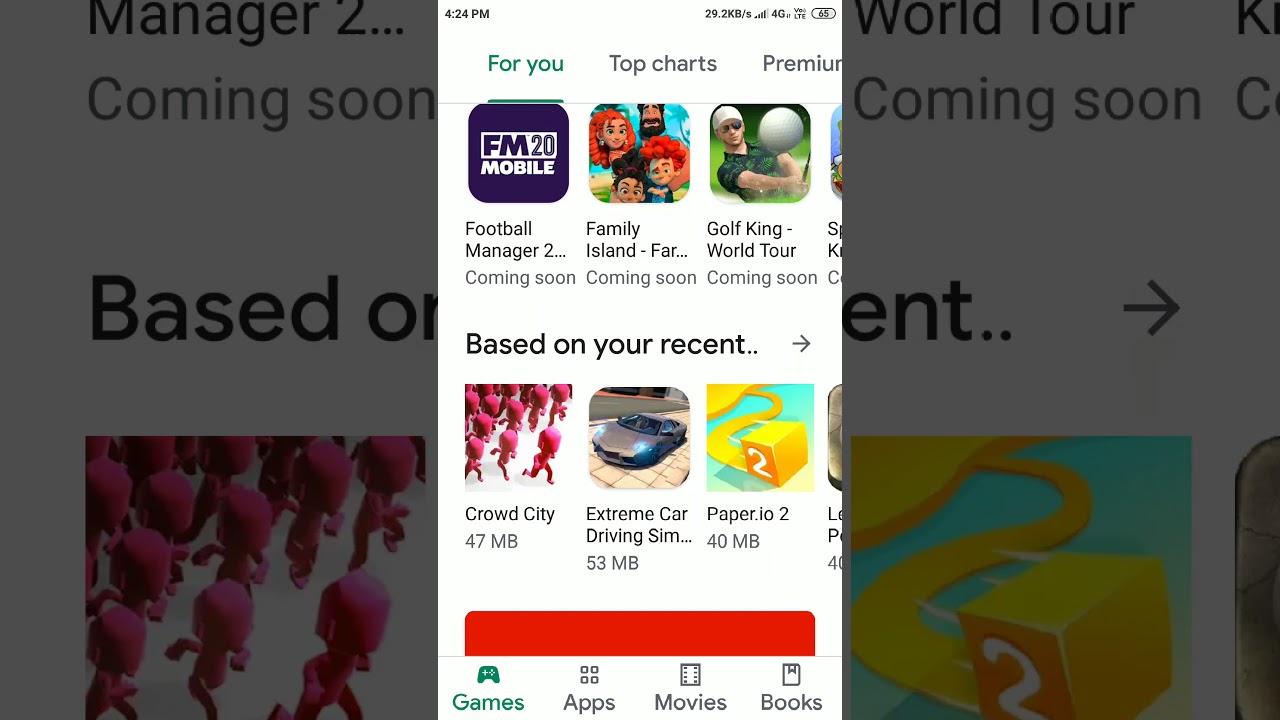The image showcases a selection of game advertisements, each featured in distinct squares. The first square on the left is purple, promoting "FM Mobile." This square also highlights that "Football Manager 2" is "coming soon." Adjacent to it, the square for "Family Island" announces another "coming soon" title, illustrated with four cartoon characters: two with red hair, one with brown hair, and another with a brown beard. Next to it, the "Golf King World Tour" square, also labeled "coming soon," depicts a man wearing a tropical shirt, white hat, and sunglasses, accompanied by a prominent golf ball.

Below these featured squares, a section titled "Based on Your Recent" is marked with an arrow. The first square here is for "Crowd City," displaying numerous small, pink characters and the text "Crowd City, 47 MB." To its right is the "Extreme Car Driving Sim" square, featuring a gleaming silver car and the text "53 MB." Continuing rightward, the "Paper.io 2" square is characterized by a yellow square and road, labeled "40 MB."

At the bottom of the image is a red rectangular bar, followed by text that categorizes content into "Games, Apps, Movies, and Books."